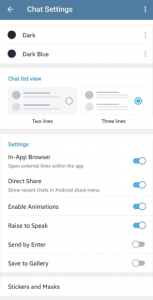Screenshot of Mobile Device Chat Settings

The image depicts a low-resolution screenshot of a mobile device's chat settings screen. The top portion of the image displays the title "Chat Settings" with a blue background, while the rest of the screen has a white background. Below the title, there are several dark circle icons labeled "Dark" and "Dark Blue," presumably for theme selection.

Further down, under the section labeled "Chat List View," there are two options: "Two Lines" and "Three Lines." The current selection is "Three Lines," indicated by a checkmark on the right.

The following settings are displayed beneath various toggle switches:

1. **In-App Browser:** Enabled - Allows opening external links within the app.
2. **Chat Share:** Enabled - Shows recent chats in the Android share menu.
3. **Enable Animations:** Enabled - Allows animations within the chat.
4. **Raise to Speak:** Enabled - Enables speaking by raising the device.
5. **Send by Enter:** Disabled - The Enter key does not send messages.
6. **Save to Gallery:** Disabled - Media is not automatically saved to the gallery.

At the bottom of the screen, under the section labeled "Stickers and Masks," there is no immediate option to toggle settings; instead, it appears tappable for further customization, as it is presented as plain text.